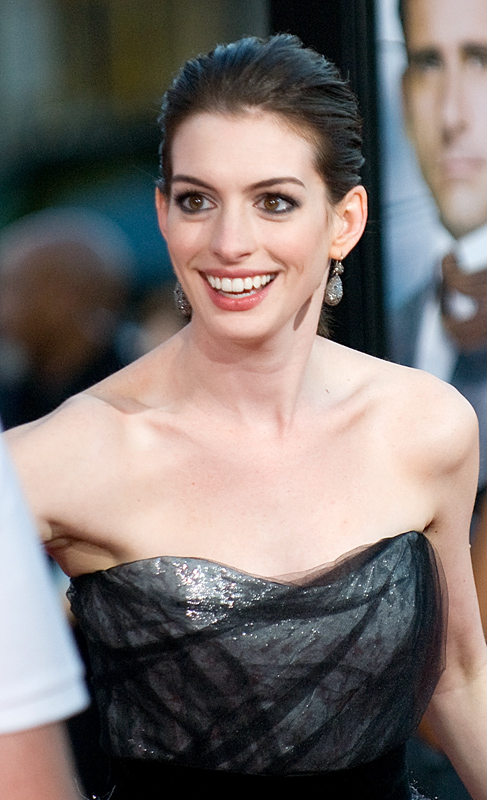In the image, Anne Hathaway is the central figure, captured outdoors, likely at a movie release event for "Get Smart." She is smiling broadly, revealing her big teeth. Anne has dark hair slicked back and is wearing drop-shaped earrings. She is adorned in a shimmery silver strapless dress overlaid with black chiffon, which contrasts with her fair skin. Her makeup is prominent, featuring red lips, and dark eye makeup. The background is blurred and features a somewhat indistinct poster of Steve Carell, identifiable by his tie, suggesting the image is indeed from the "Get Smart" red carpet. There is no visible text in the image, and it includes a mix of colors like black, gray, white, tan, red, and pink. Her thin shoulders and arms are also notable, and there appears to be a white brooch over one arm. The overall setting is characterized by a brownish blur, likely indicating the event's atmosphere.